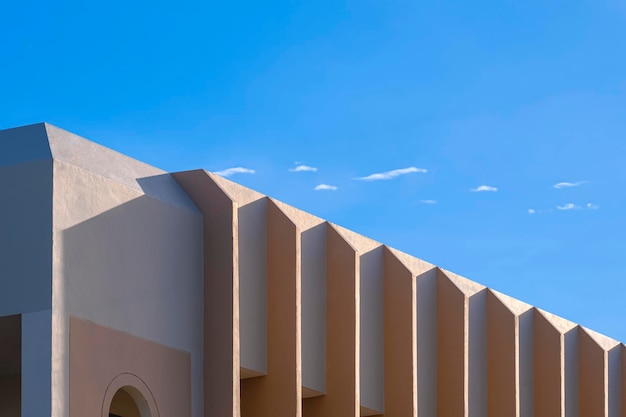The image captures the upper portion of a modern-style building against a clear blue sky with a few thin, wispy clouds. The building, composed primarily of sandy-colored or beige concrete, features distinct textures and shadows that give it a 3D, comb-like appearance. Along the walls, light brown, column-like structures protrude, adding depth and design complexity. The facade includes an arched window accented with light brown shades and several square windows nestled in the recesses, providing contrast. The brightly lit day enhances the play of shadows along the building's textured surfaces, emphasizing its architectural intricacies.